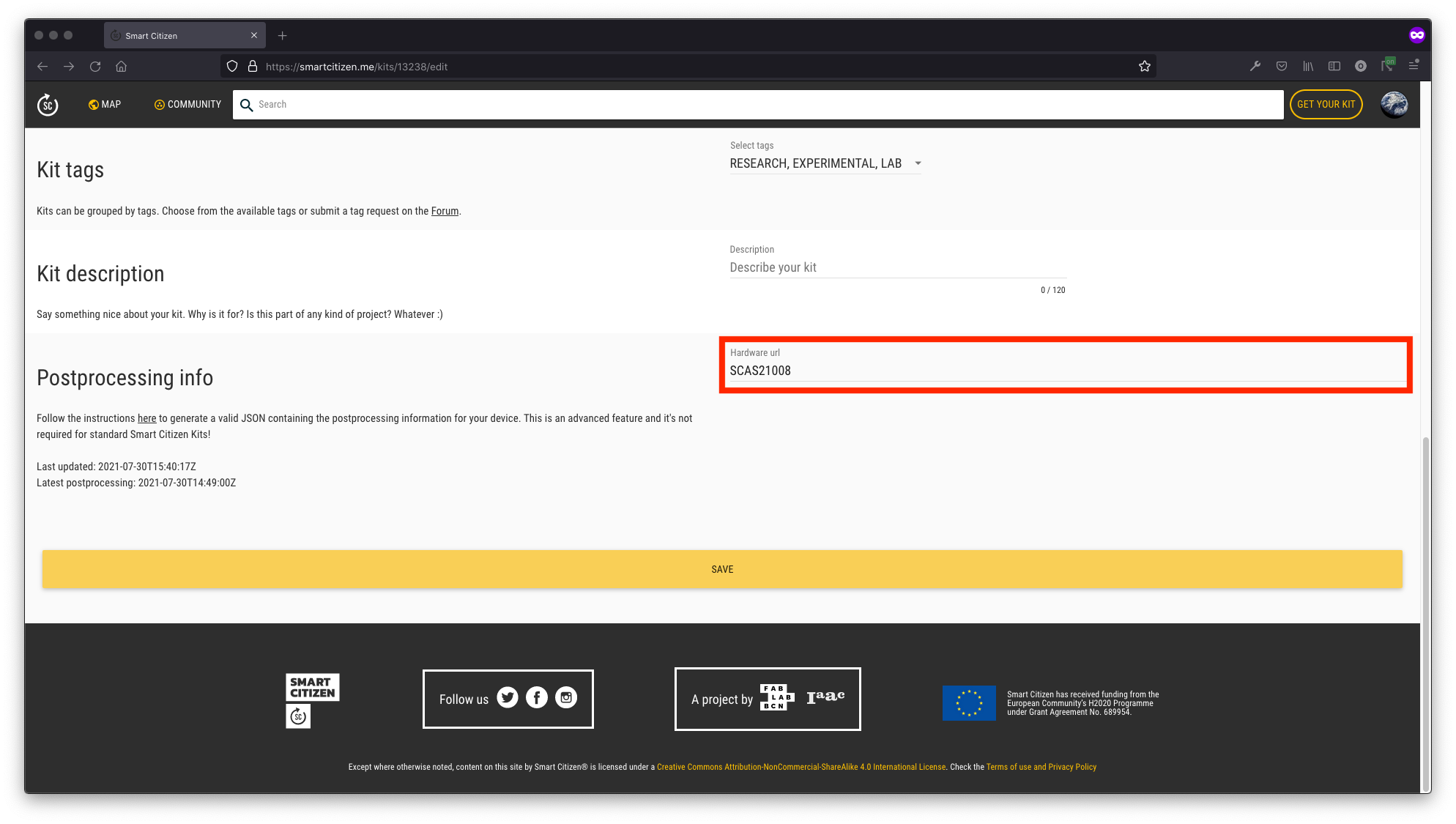This image showcases a computer screenshot featuring a webpage interface. At the very top, the presence of a browser is evident with the visible search bar and multiple open tabs. In the upper left corner of the webpage, the words "Map" and "Community" are displayed prominently. Just below these terms, the label "Kit Tags" is visible, followed by a small, hard-to-read description in tiny letters. Adjacent to this section, there is an indication of "End Tags" and the phrase "Research Experimental Lab," accompanied by a dropdown menu.

Below "Kit Tags," on the left side, the page features the heading "Kit Description" with a prompt that says, "Say something nice about your kit. What is it for, is this a great part of any project, whatever," ending with a smiley face. To the right of this, a section titled "Description" includes a line that prompts users to "Describe your kit."

Further down, the left side displays "Post Processing Info" with several lines of text that are notably tiny and hard to decipher. On the right side of this section, there’s a column containing a number outlined in a red text box. The purpose and details of these numbers are unclear due to their minute size.

At the very bottom of the interface, a large yellow button with the text "Save" stands out, inviting users to finalize their input.